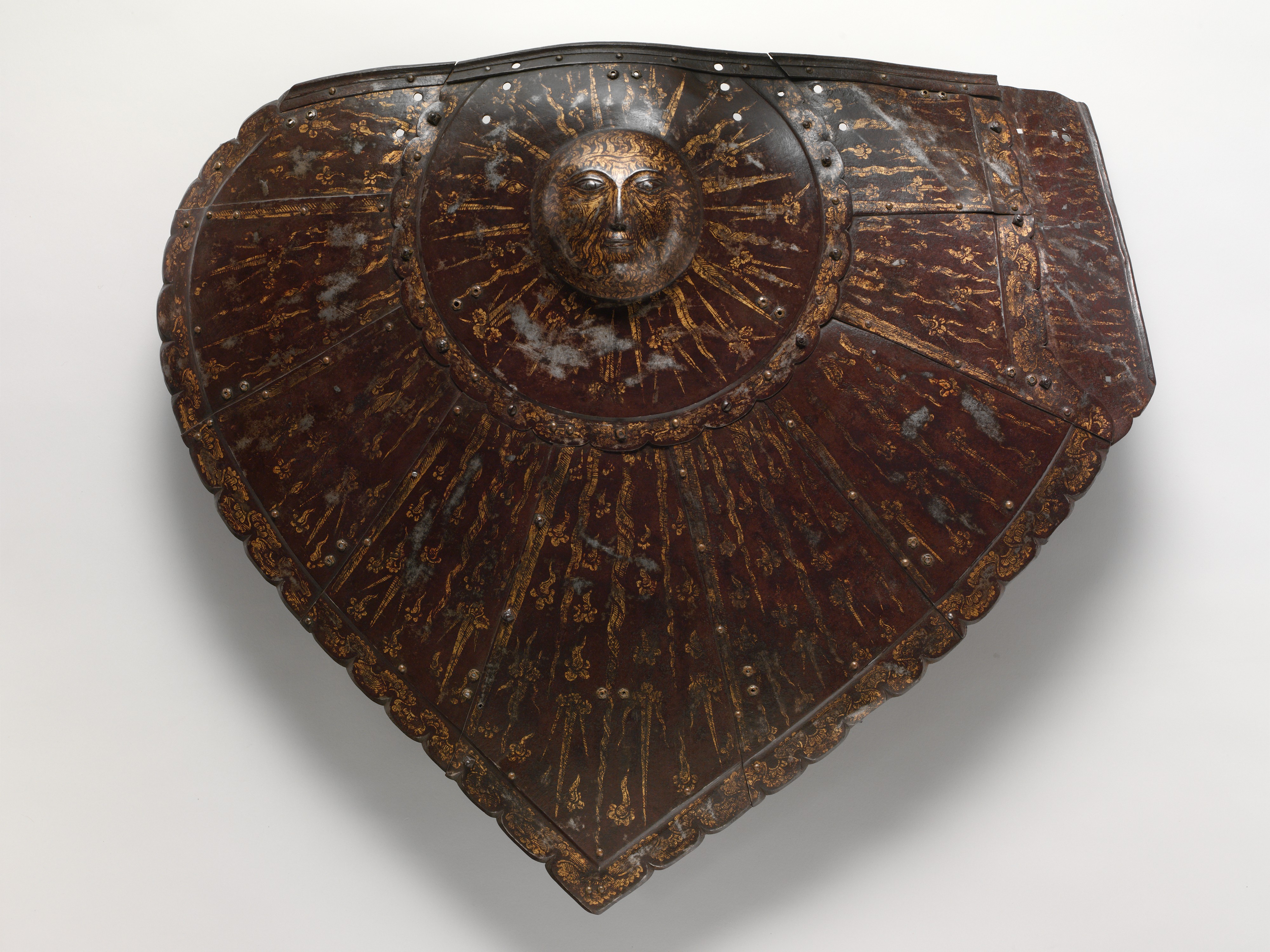The photograph features an intricately designed shield, resembling an upside-down arrowhead or teardrop, aligning with a heart shape, characterized by two curved sides merging at a pointed bottom and a flat yet undulating top edge. The shield's primary surface displays a prominent sun motif at its center, meticulously carved to depict a face with two eyes, eyebrows, a nose, and a small mouth. Golden, semi-thick wavy lines, reminiscent of sunbeams, radiate outward from the central sun, stretching across the shield's surface. Its border is adorned with a delicate, wavy line pattern that mirrors an intricate design along the shield's edge. A vertical, rectangular element, sharing the same gold outline and intricate design as the bottom border, extends from the shield's top. Dominated by hues of brown, gold, tan, gray, black, and white, the artistic shield occupies the central position within a square composition, set against a plain white background.